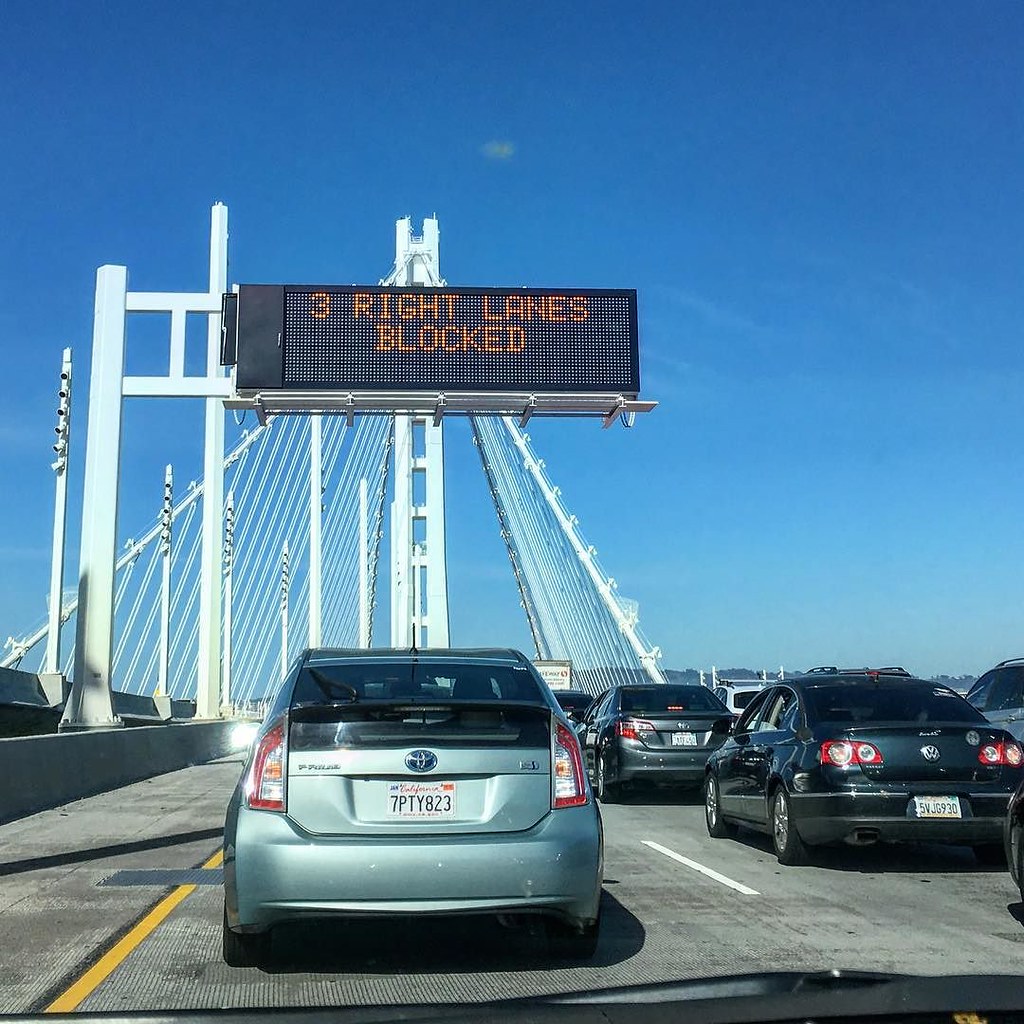In this photograph, taken from the perspective of a vehicle on a bridge, the scene vividly captures a standstill traffic jam. Numerous cars, including a noticeable silver car and several black vehicles, are tightly packed and immobile, indicating heavy gridlock. The backdrop features the upper structure of the bridge against a clear, azure sky, suggesting the photo was taken on a bright, sunny day. Dominating the scene is an illuminated street sign overhead, which reads "Three right lanes blocked," offering a clear explanation for the traffic congestion. This detailed image portrays the frustrating pause in the flow of vehicles due to a significant lane closure ahead.